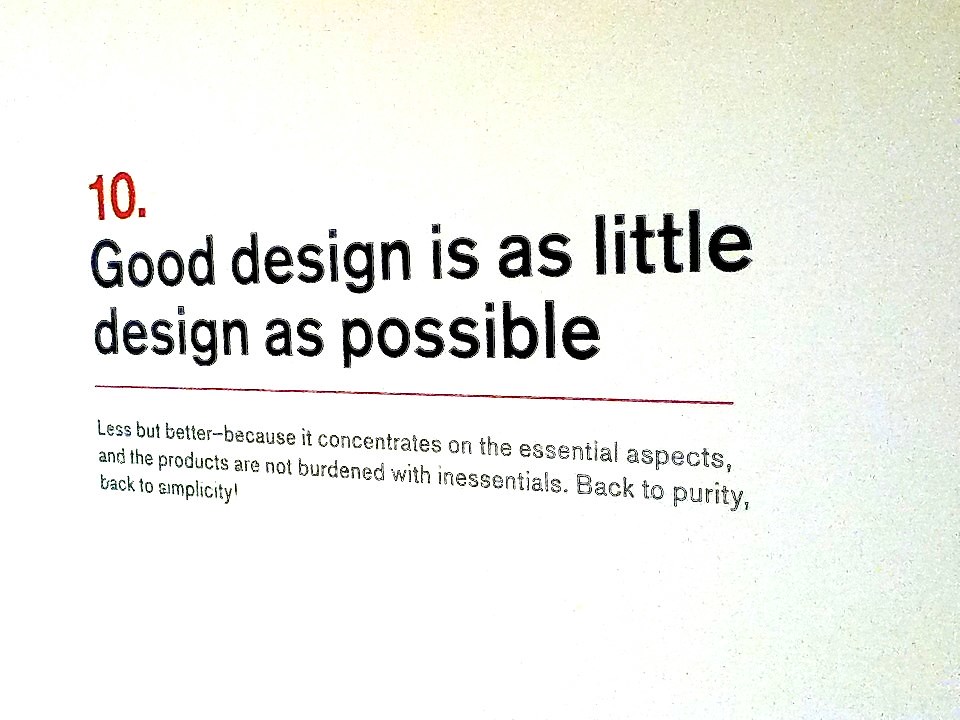The image appears to be a slide or placard, capturing a minimalist design ethos. At the very top is the number "10" printed in bold red, presumably indicating its sequence in a larger series. Below this, in prominent black text, is the statement: "Good design is as little design as possible." This central tenet is underscored by a thin horizontal line in red. Beneath this line lies a paragraph in smaller black text, articulating a philosophy of simplicity: "Less but better – because it concentrates on the essential aspects, and the products are not burdened with inessentials. Back to purity, back to simplicity!" The background of the slide is predominantly white, with subtle hints of very light green on the right edge, adding a touch of color to the otherwise stark design. The image is slightly angled, causing the right side to appear marginally larger than the left, with a grainy texture around the edges due to the lighting.